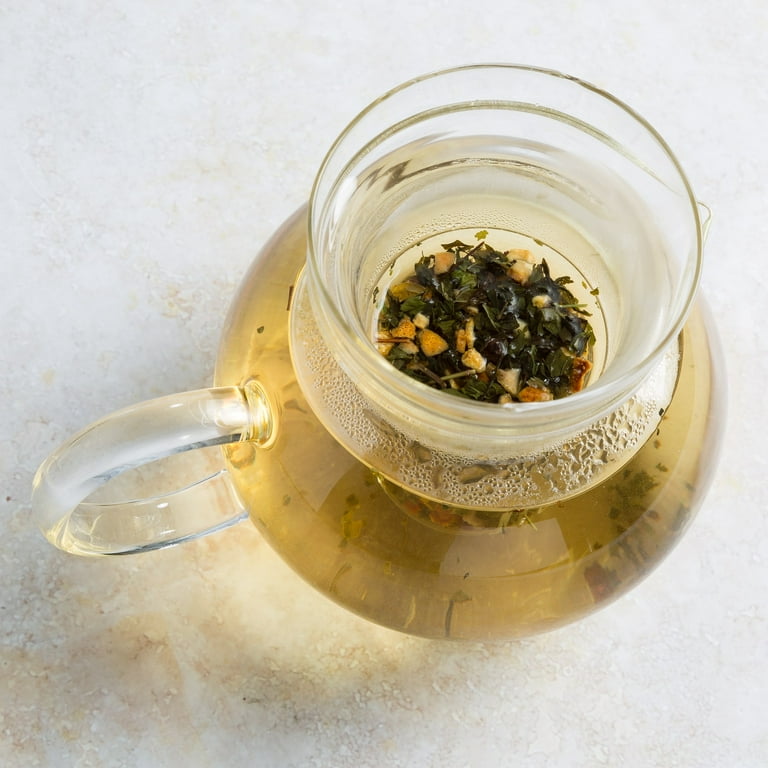The photograph showcases a large, round, and translucent glass teapot with an integrated infuser area on top, perfect for steeping tea leaves and spices. The teapot is bulb-shaped, with a substantial, clear handle positioned on the left. It sits on a pristine white marble countertop, illuminated by sunlight streaming from the top right, which creates a warm glow on the surface. The tea inside the teapot has steeped to a light amber hue, though some tea leaves have filtered through, indicating imperfect filtration. Steam bubbles cling to the inner walls of the teapot, suggesting recently added hot water. The combination of the elegant glass design and the rich blend of ingredients makes for a visually appealing and functional piece, ideal for tea lovers.